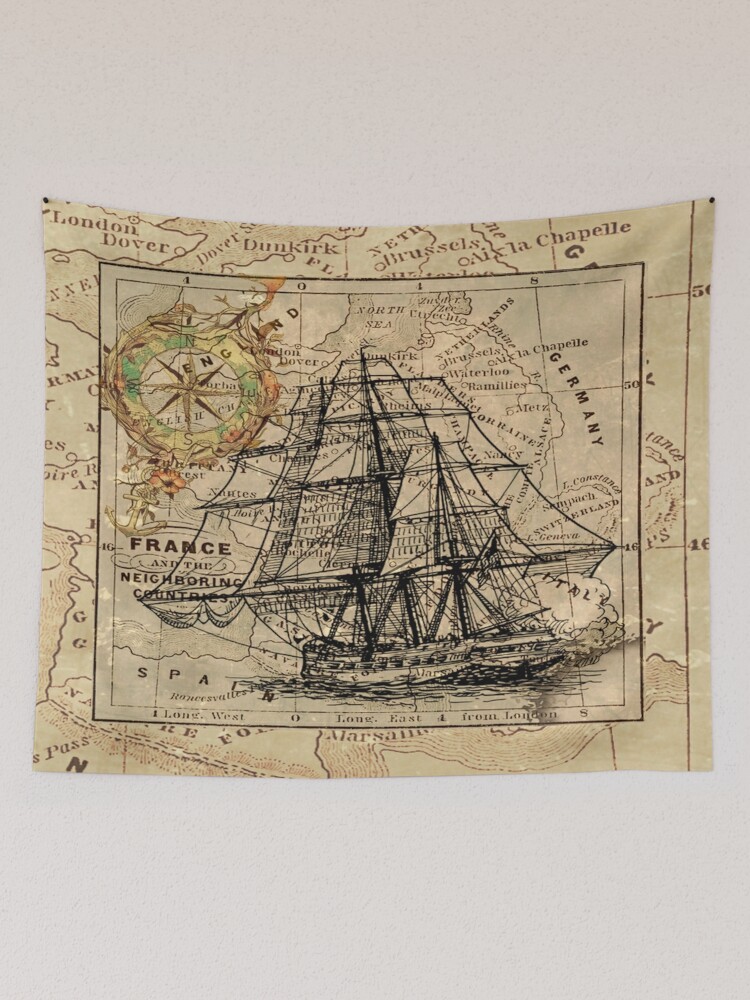The image depicts a vintage, textile-style map of Europe, draped against a faded grayish-pink wall, secured at the top corners with two push pins. The map, which has a tan, cloth-like appearance, showcases various regions including Germany, England, France, and Spain. At the top left, notable locations such as London, Dover, Dunkirk, and Brussels are marked. Central to the map, an ornate square frames a prominent black-and-white illustration of a large sailing ship with towering masts, partially obscuring the countries beneath it. A colorful compass featuring green and yellow hues, with a star or diamond pattern in the middle, is positioned at the upper left corner of the square, pointing west and east. The combination of the detailed cartography and the intricate ship design creates a striking, layered visual effect.